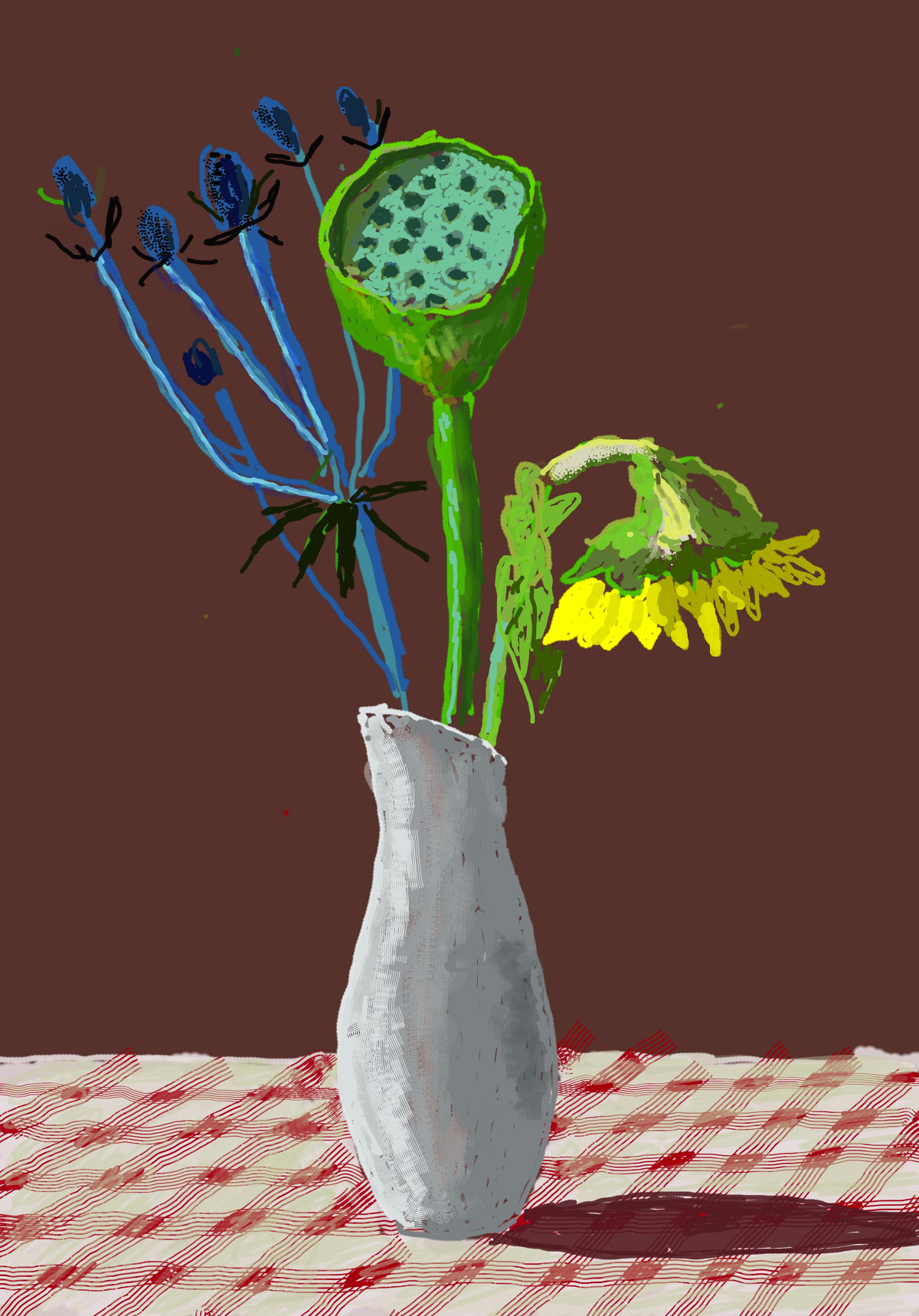In this striking digital illustration, a tall, slender white clay vase dominates the scene, set against a solid maroon backdrop. The vase is perched on a table adorned with a red and white checkered tablecloth, featuring a pattern of crisscrossing stripes forming a combination of red and white squares. The composition captures an abstract interpretation of flowers, with various blooms extending from the vase. Among them are sprigs of blue flowers with long, thin stems and small oval-shaped petals, clustered mainly in the upper left section. A central green stalk resembles a cucumber, and on the right, a yellow sunflower droops downward, its head bent toward the table. The overall effect is a masterful blend of detailed floral elements and abstract artistry, casting intricate shadows and inviting closer inspection.